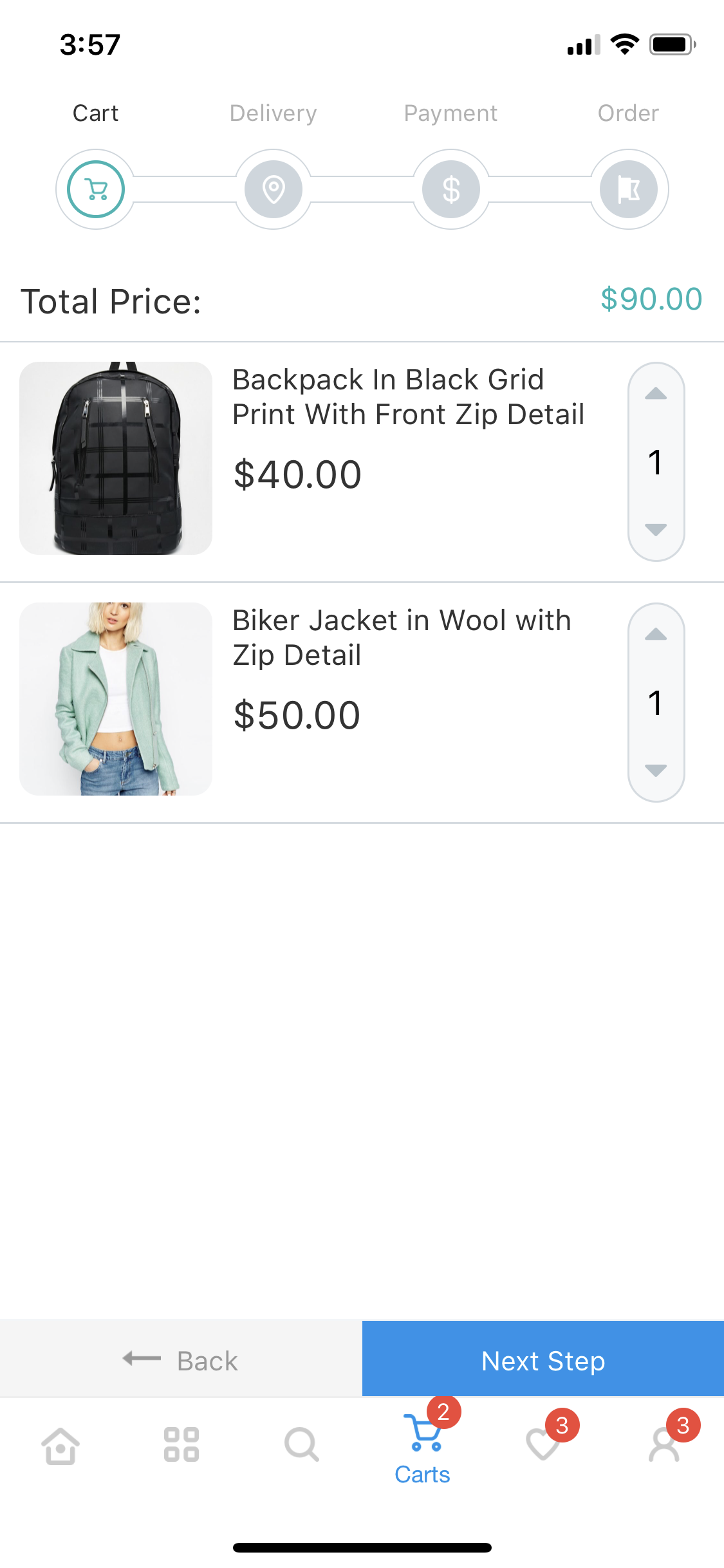The image is a detailed screenshot of a shopping cart from an online shopping website. At the very top of the screen, the cell bar displays the current time on the top left, and on the top right are the cell phone signal strength, Wi-Fi connectivity icon, and battery level indicator.

Directly below the cell bar, there are four navigational categories labeled "Cart," "Delivery," "Payment," and "Order." Each category is represented by a circular icon connected by a line. The "Cart" category features a shopping cart icon, "Delivery" has a location pin symbol, "Payment" displays a dollar sign, and "Order" is marked with a flag icon.

Underneath these categories, the total price of the items in the cart is shown on the right side of the screen, amounting to $90. Below this, the items in the cart are listed with accompanying images. 

The first item is a black backpack with a black grid pattern and front zip detail, priced at $40. To the right of its description, the quantity is indicated as one.

The second item is a woman's teal biker jacket made of wool, featuring a zip detail, priced at $50. Similarly, the quantity is indicated as one on the right.

At the bottom of the screen, there are two buttons: a "Back" button in light gray and a "Next Step" button in blue. 

Furthermore, at the very bottom of the screen is a navigation bar featuring a home icon, a grid-like four-box icon, a search icon, and a cart icon in blue with a red circle displaying the number "2" for the items in the cart. Additionally, there is a heart icon with a red circle showing the number "3," and a person icon with a red circle also indicating the number "3."